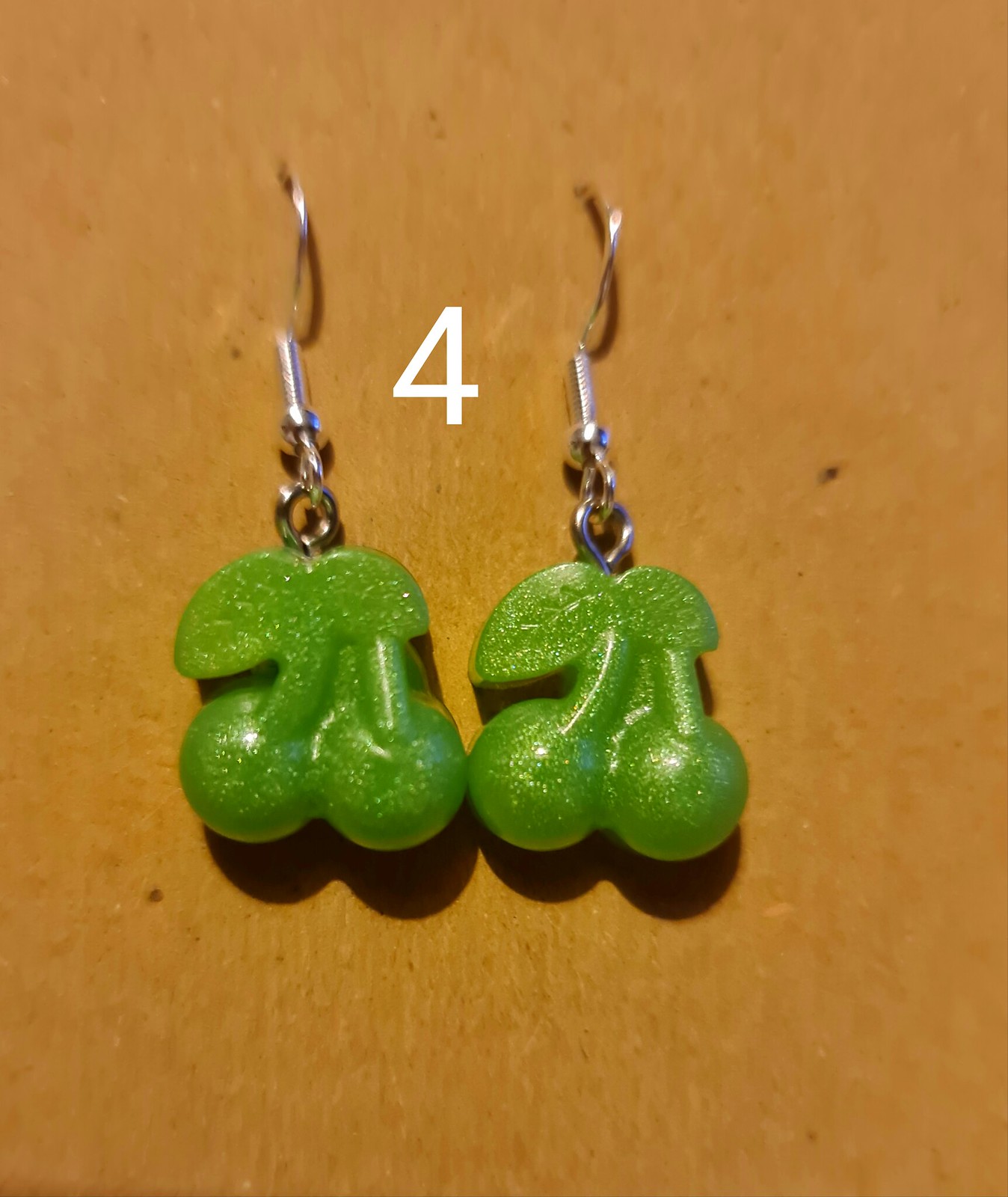This detailed photograph showcases a pair of identical earrings displayed against a pegboard backdrop, which is brown in color, possibly wooden. Each earring features a silver clasp designed for pierced ears, detailed with a spring and hook mechanism. Dangling from these clasps are glossy, green plastic elements sculpted to resemble a pair of cherries, complete with twigs and leaves, enhancing the realistic and playful design. Positioned centrally between the two earrings is the number 4, elegantly written in white. The pegboard background suggests that these earrings might be presented for sale on platforms such as Etsy or eBay, with additional holes visible in the board, indicating past displays of other earrings.